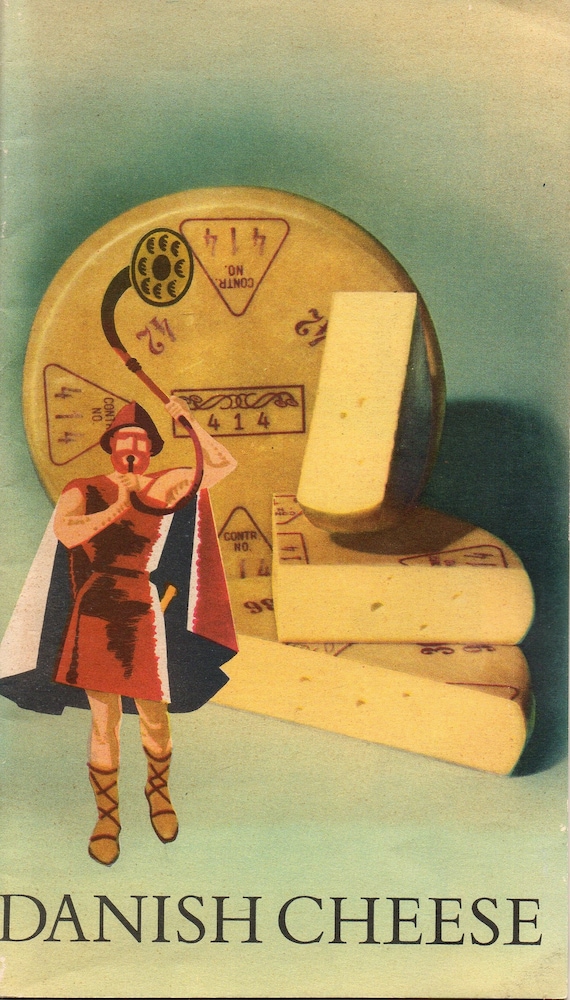The poster is an advertisement for Danish cheese, prominently featuring a bold, black, all-caps caption at the bottom that reads "DANISH CHEESE." In the background, several blocks of cheese are displayed, including a full round cheese wheel, a half-wheel, and quarters of the wheel, each meticulously stacked and arranged. The cheese prominently features the numbers "414" along with intricate symbols and insignias.

Foregrounded in this illustrated scene is a character resembling a Danish warrior, possibly a Viking. The warrior has a striking red beard and dons a hat with a distinctly Danish appearance. He is clad in a detailed outfit featuring a cloak with a dark blue inside and a red and white exterior. His attire includes a one-piece skirt-like garment with a belt, which complements his brown crisscross-strapped sandals. Additionally, he wears old-fashioned armor with shades of brown.

The warrior is depicted blowing into a unique, elongated horn or pipe that curves back on itself, resembling an ancient musical instrument with a bell-like end similar to a trombone or an Alpenhorn. This fantastical, illustrative combination sets the scene for an eye-catching and thematic advertisement for Danish cheese.